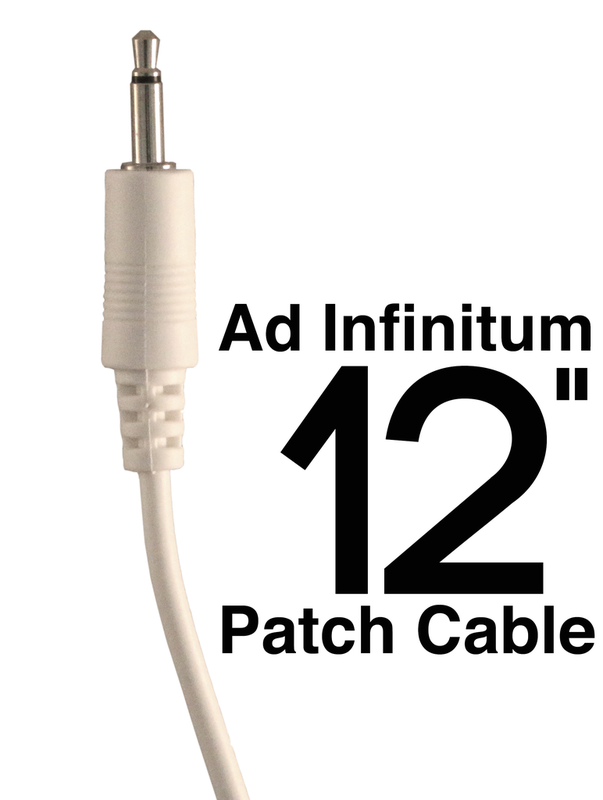This is a detailed close-up image of an electronic device on a pure white background. On the left side of the frame, a white cable runs upward from the bottom left corner. The cable features a ridged white cylinder transitioning into a smooth white cylinder with small darker ridges in its center. At the top of the smooth cylinder is a silvery disc connected to a long silver cylinder, which ends in a slightly flared silver piece at the very top. Positioned to the right of the cable, in large bold black text, are the words "ad infinitum." Directly beneath this, in even larger black text, is "12 inches," and near the bottom of the frame, in medium-sized black text, it says "patch cable." The image serves to describe the 12-inch patch cable by "ad infinitum," highlighting its white, plastic rubber appearance and distinctive silver connector end.